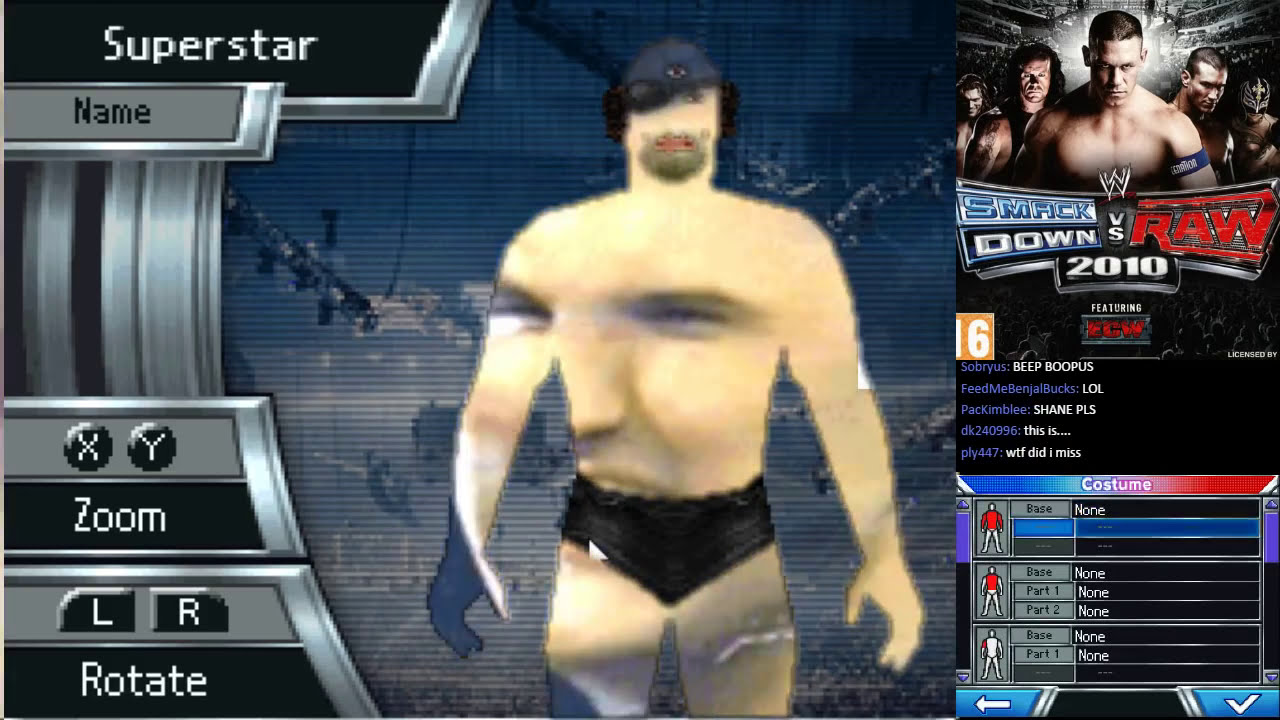The image is a detailed screenshot from the computer game "Smackdown vs. Raw 2010 featuring ECW." In the center, there is a cartoon depiction of a shirtless wrestler wearing black trunks, with a superimposed face of a man squinting and screaming. This character is surrounded by an elaborate backdrop featuring planes and a skybot.

On the top left, "Superstar" is displayed in white text against a black background, with a gray panel below it featuring the label "Name." The bottom left corner shows game controls: "X" and "Y" buttons for zooming, and "L" and "R" buttons for rotating.

To the right, there is a panel highlighting a shirtless wrestler with short hair and an armband, positioned in front of several menacing wrestlers. Beneath this image, the text "Smackdown vs. Raw 2010" is displayed above the phrase "featuring ECW." Below this, there are options to customize the wrestler's costume. This area also includes what appears to be a live chat, possibly indicating the game is being live-streamed.